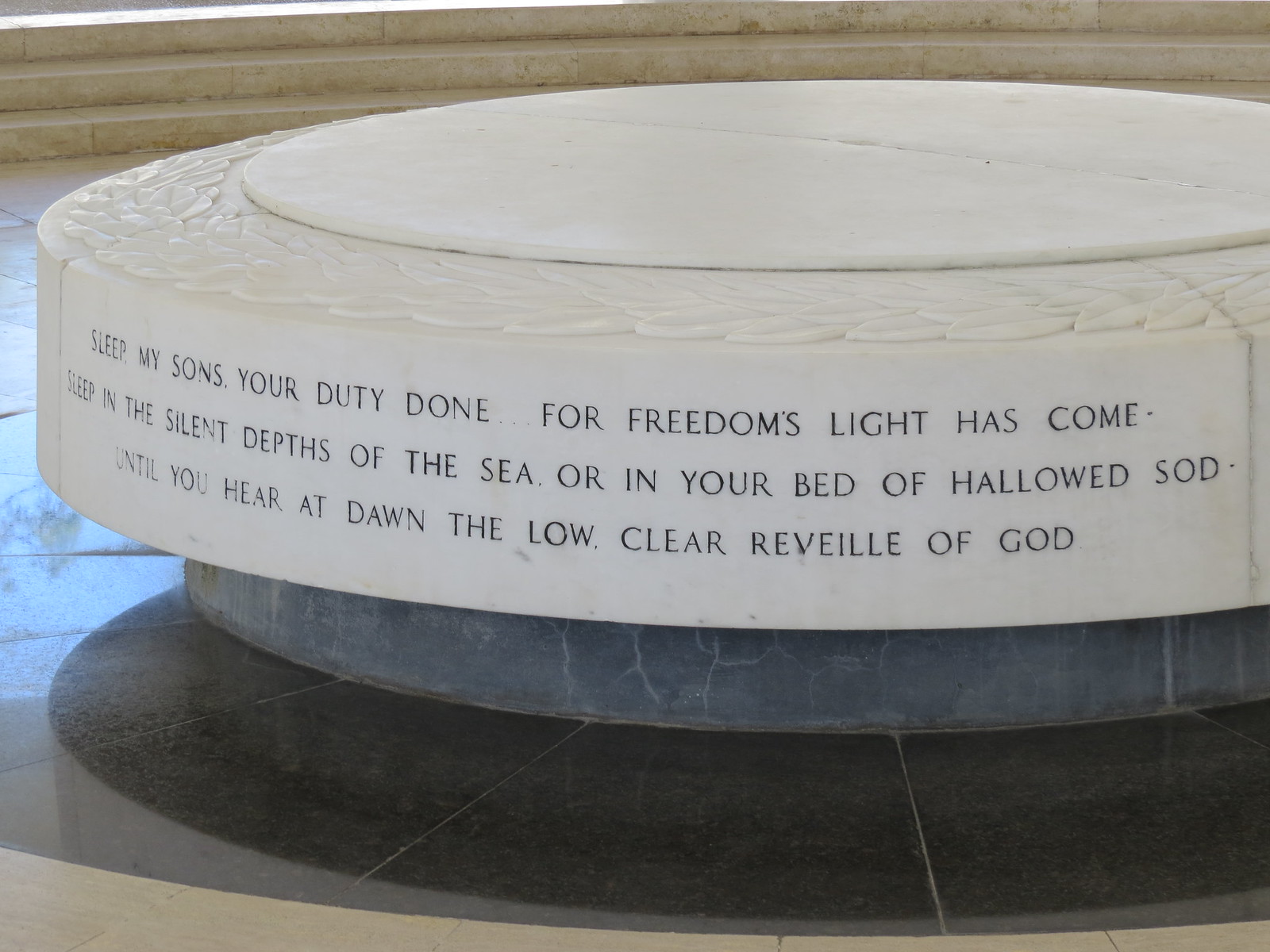This is a color photograph of a military monument likely located indoors, possibly in a museum or a memorial area that could also resemble a fountain. The centerpiece is a white, disc-shaped sculpture made from white marble, resting on a smaller, round gray marble base. The inscription, intricately chiseled in capital black letters in a serif font, probably Garamond, reads: "Sleep, my sons, your duty done, for freedom's light has come. Sleep in the silent depths of the sea, or in your bed of hallowed sod, until you hear at dawn the low, clear revelry of God." The surrounding floor is made of concrete, and the monument is likely in a central position, signifying its importance and reverence for fallen soldiers and sailors.